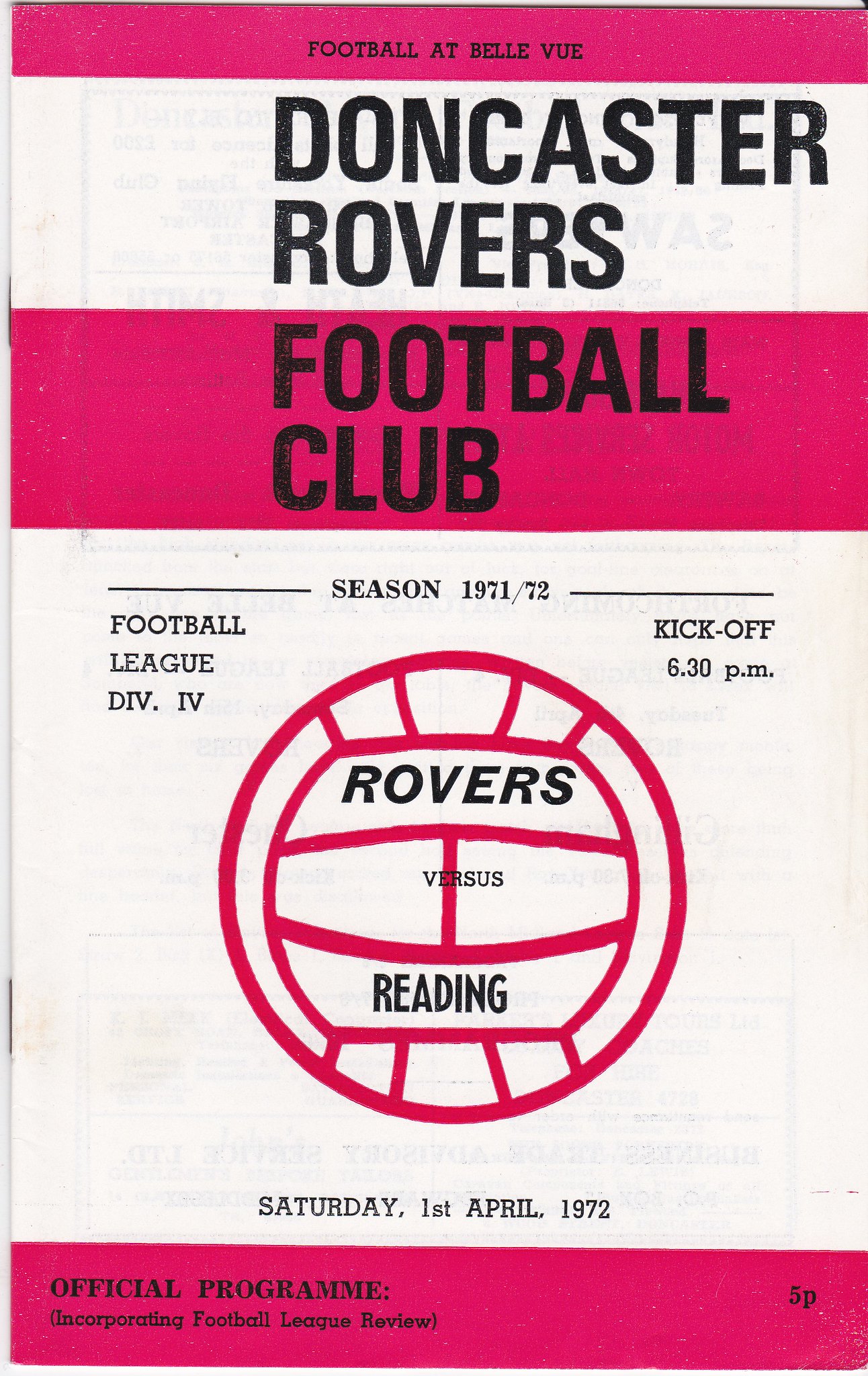This image is the cover of an official program for a football match, showcasing a design from the 1971-72 season. The cover features a striking pink and white color scheme. At the top, on a pink background with small black letters, it reads "Football at Bellevue." Below this, in larger black letters on a white stripe, it displays "Doncaster Rovers." A pink stripe follows, with "Football Club" written in black. The central section of the cover prominently features the match details: "Rovers vs Reading," set within a graphic of a pink soccer ball on a white background. Additional information includes the season (1971-72) and the division (Football League Division 4) arranged in Roman numerals. The kickoff time is 6:30 p.m. on Saturday, April 1st, 1972. Underneath, a pink banner declares this as the "Official Program," incorporating "Football League Review" for 5 pence. The bottom corner notes the price as 5p, and the cover also displays some faint images of staples along the left binding, indicating a booklet form.